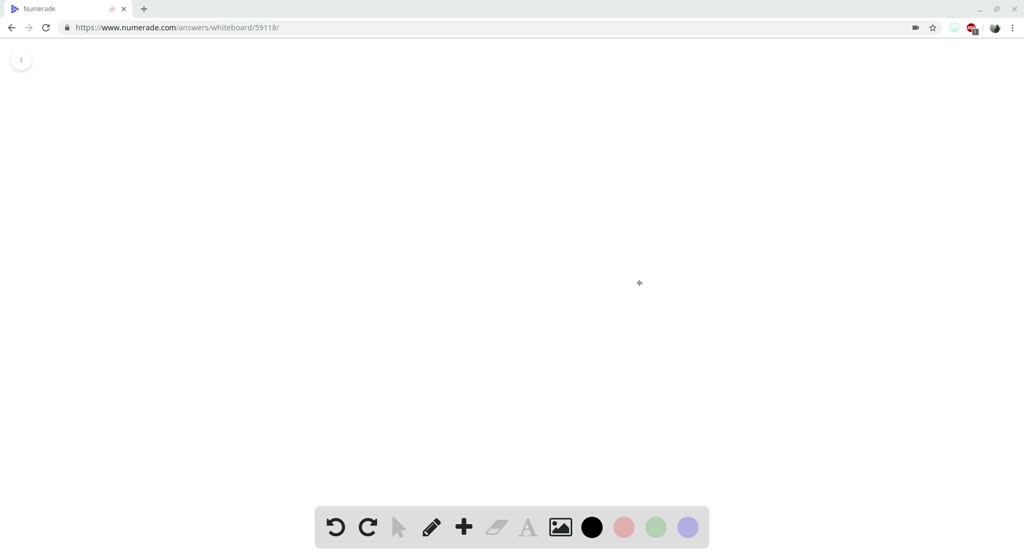The image depicts a web browser window, likely Google Chrome, with a rectangular aspect ratio that is approximately 50% wider than it is tall. At the top of the window is the familiar Windows taskbar, featuring the minimize, maximize, and close buttons in the upper right corner, with the maximize button represented by overlapping squares.

On the left side of the browser, a single tab is open, marked by a dark blue right-pointing triangle and a small 'X' for closing the tab. To its right is a plus symbol allowing the user to open a new tab. The address bar below the tabs includes a left arrow (back button) colored solid black, a grayed-out right arrow (forward button), a refresh icon depicted as a nearly complete circle with an arrow at the one o'clock position, and a lock symbol indicating a secure connection, followed by the URL.

The majority of the browser's viewport is white, save for a gray toolbar at the bottom center. This toolbar contains various editing tools, including an undo button, a pencil icon for drawing or writing, a plus symbol for adding elements, and options to insert images, among others.